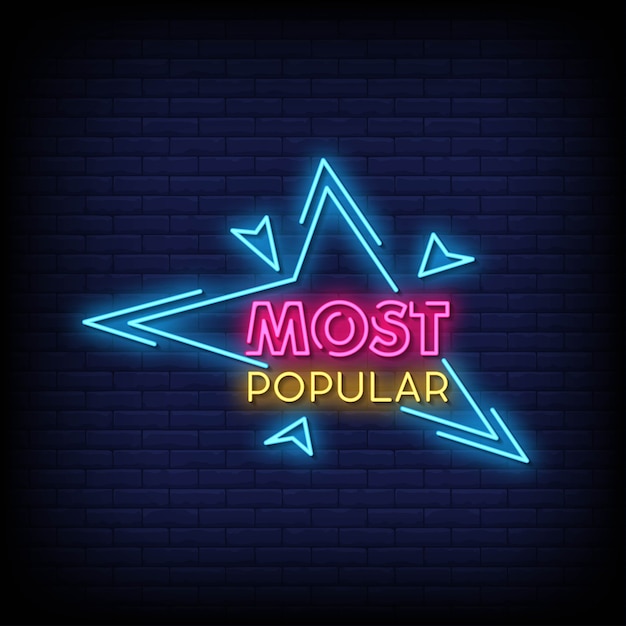The image showcases a neon sign affixed to a dark, possibly navy blue or black, brick wall, which fades into darkness at the edges. The main feature of the sign is a large, angular teal arrow pointing towards the center, where the words "MOST POPULAR" are prominently displayed. "MOST" is written in hollow, bubble-like pink neon uppercase letters, while "POPULAR" is in solid yellow uppercase letters. Surrounding the main arrow are three smaller arrows, also outlined in neon, directing attention towards the central text. The sign’s illumination slightly lights up the surrounding brick wall, creating a stark contrast against the otherwise pitch-black background. This detailed, vibrant neon design makes the message "MOST POPULAR" visually striking on the dark backdrop.